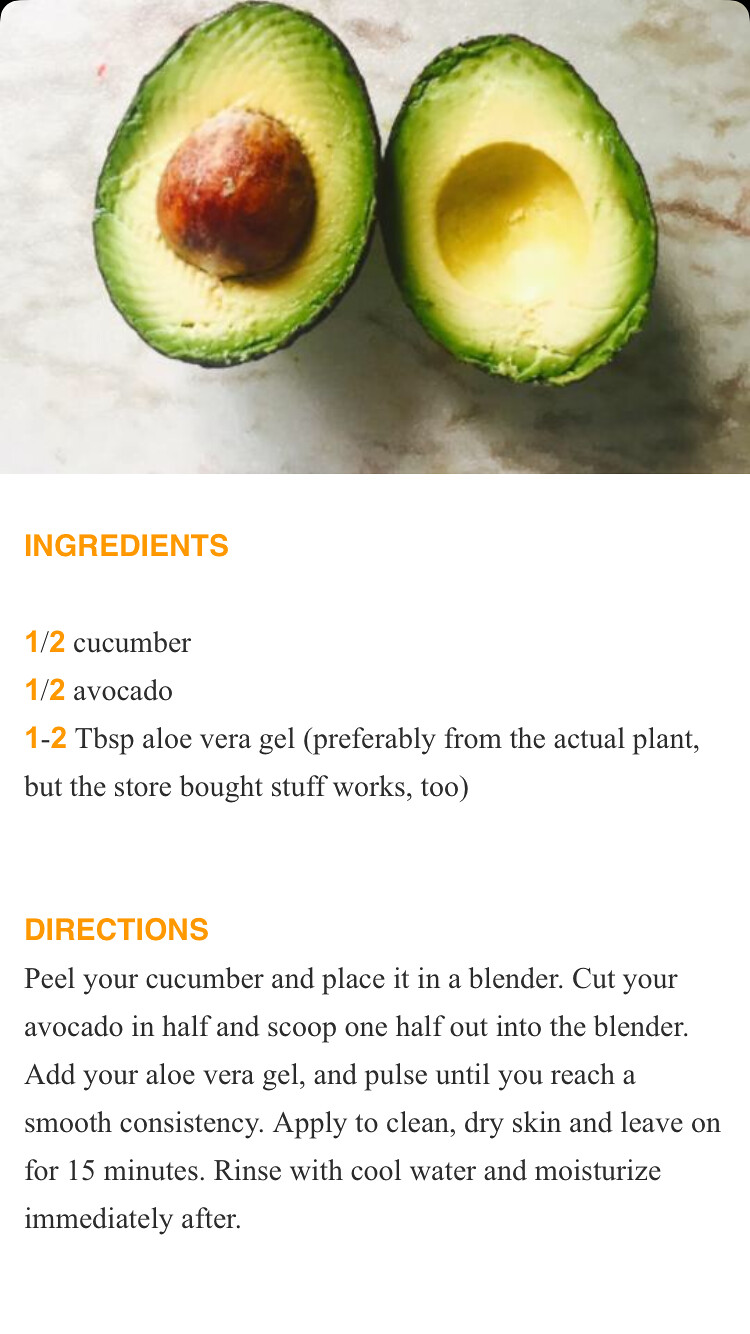The image is a screenshot of a website recipe for creating a skincare gel using natural ingredients. At the top, there is a prominent photograph of an avocado cut in half, with the left half containing the pit and the right half being pitless. The visual is set against a white background with subtle gray and brown hues mingling in the countertop. Below the image, the recipe details start with an "Ingredients" list, which includes half a cucumber, half an avocado, and one to two tablespoons of aloe vera gel - preferably fresh from the plant, though store-bought gel is acceptable too. Following this is the "Directions" section, printed in orange text, while the rest of the instructions are in black. It guides the user to peel the cucumber and place it in a blender, scoop out half of the avocado into the blender, add the aloe vera gel, and blend until smooth. The final product should be applied to clean, dry skin, left on for 15 minutes, rinsed off with cool water, and followed by immediate moisturizing. This recipe highlights its use in skincare rather than as a food item.